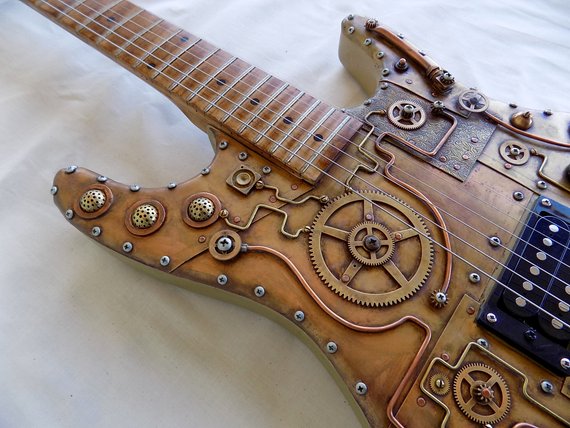The image is a detailed close-up of a steampunk-themed electric guitar, showcasing the midsection up to the middle of the top part of the instrument. The guitar features an ornate, intricate design with six strings gradually widening towards the bottom. The body is adorned with a myriad of steampunk elements, including several gears and round mechanical components, both small and massive, giving it a distinctive industrial look. Brass tubing leads to sprockets and screws, securely fastening various pieces of metal and plates, adding to the complex aesthetic. The guitar's decoration includes copper or brass domes with holes drilled through them, assorted bolts, and a hyper-stylized arrangement of wires across its design. Various screws, estimated to be around 10 to 15 or more, are placed meticulously along the edges and surfaces, further enhancing the steampunk vibe. The predominant colors of the guitar are brown, white, and silver, with some black elements in the middle part, featuring silver circles. The entire setup rests on what appears to be a white tablecloth, giving a sharp contrast to the guitar's elaborate design.